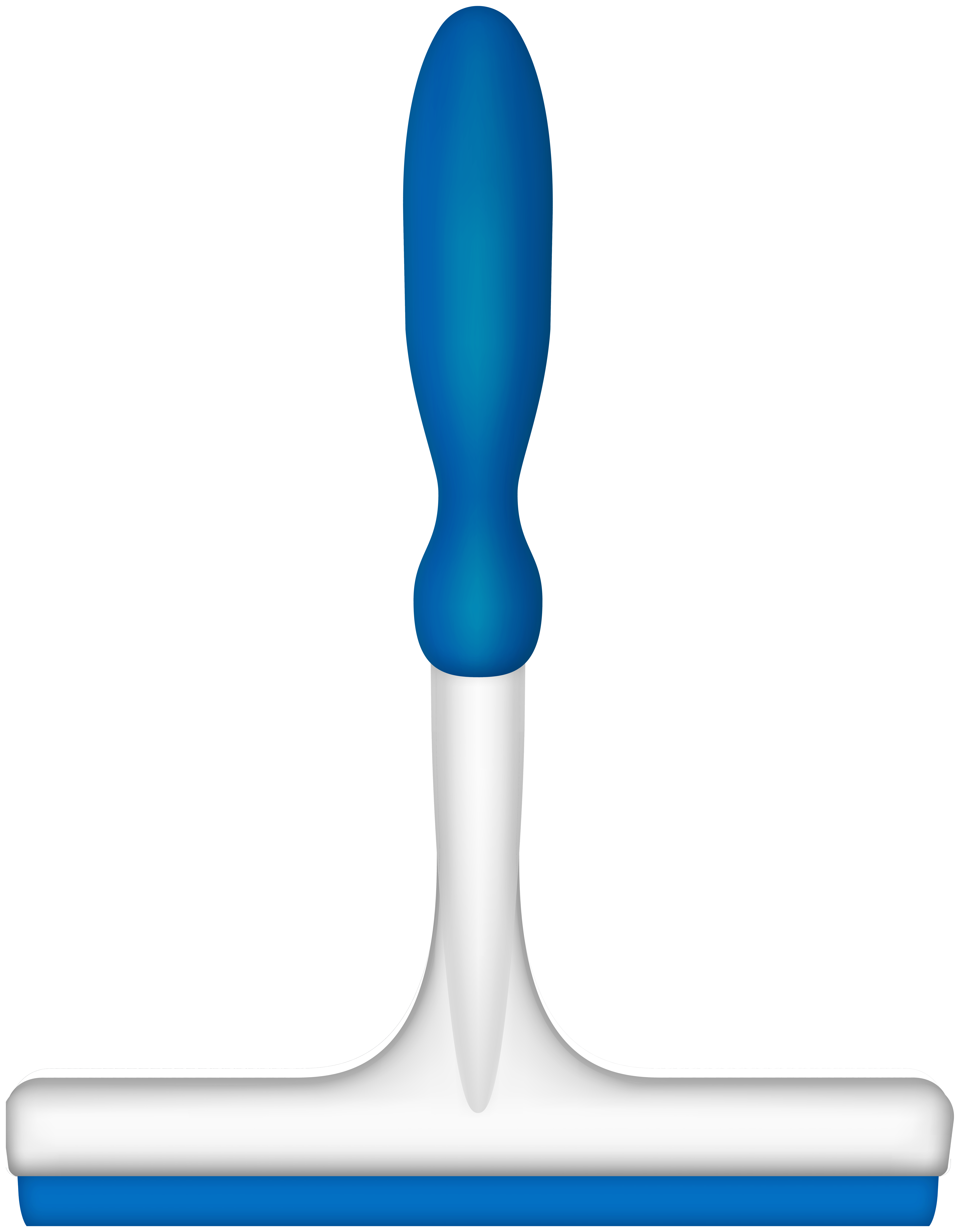This image is a simple piece of vector art depicting a squeegee set against a completely white background. The squeegee features a white body with a blue grip and a blue blade. The blue handle at the top of the image has an hourglass shape, starting wider at the end and tapering towards the center before flaring out again where it meets the white portion of the handle. The handle is capped with a gradient that transitions from a darker blue at the edges to a lighter blue towards the center, giving it a slight 3D effect. Below the handle, the white body of the squeegee narrows into a T-shape where the horizontal segment meets the vertical handle. A distinct raised ridge in the form of a small V is present on the white portion near the base. The blue rubber blade of the squeegee, positioned horizontally, runs along the bottom of the device, completing its utilitarian design.